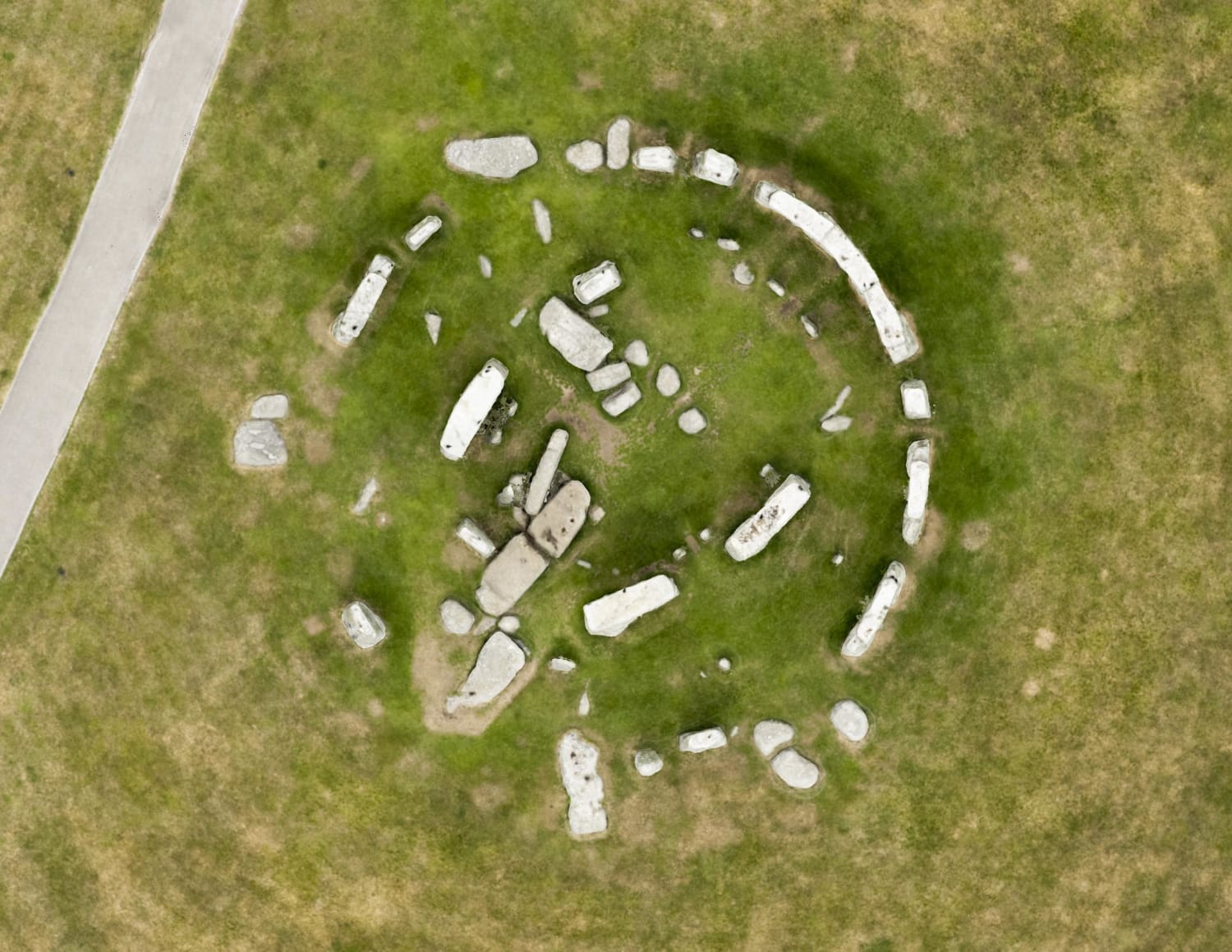This aerial photograph captures the iconic Stonehenge monument from directly above, showcasing its distinctive semi-circular layout of massive stones. The green grass below features patches of brown, indicating areas of wear or sparse growth, particularly thicker around the stones. The outer rim of the semi-circle has various stones, with larger stones forming structures where two vertical stones support a horizontal one atop. Inside this semi-circle, additional stones are scattered, hinting at what was once a complete circle. In the background, a lightly trafficked road, appearing as a grey diagonal line, cuts through the upper left corner of the image, emphasizing the isolation of this ancient site. The stones, predominantly hues of white and grey, stand starkly against the grassy and earthy backdrop. No people or text are visible in this serene and historic landscape.